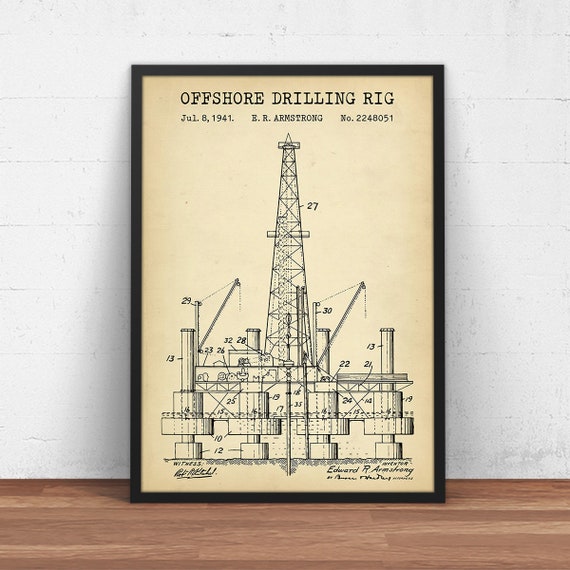This is a detailed photo of a framed blueprint titled "Offshore Drilling Rig," dated July 8, 1941, by E.R. Armstrong, number 2248051. The print, which has aged into an off-white or beige hue, is enclosed in a black frame. It rests on a brown wooden floor and leans against a white stone wall. The blueprint features a meticulous diagram of an oil rig, with various parts labeled by numbers. At the base, it depicts four pillars set in water, spaced 12 feet apart. The pillars rise to different heights with varying gaps, showing the engineering intricacies. The main structure includes a tall tower and extending arms, detailed in gray and white. The bottom right corner bears the name Edward R. Armstrong, identified as the inventor.